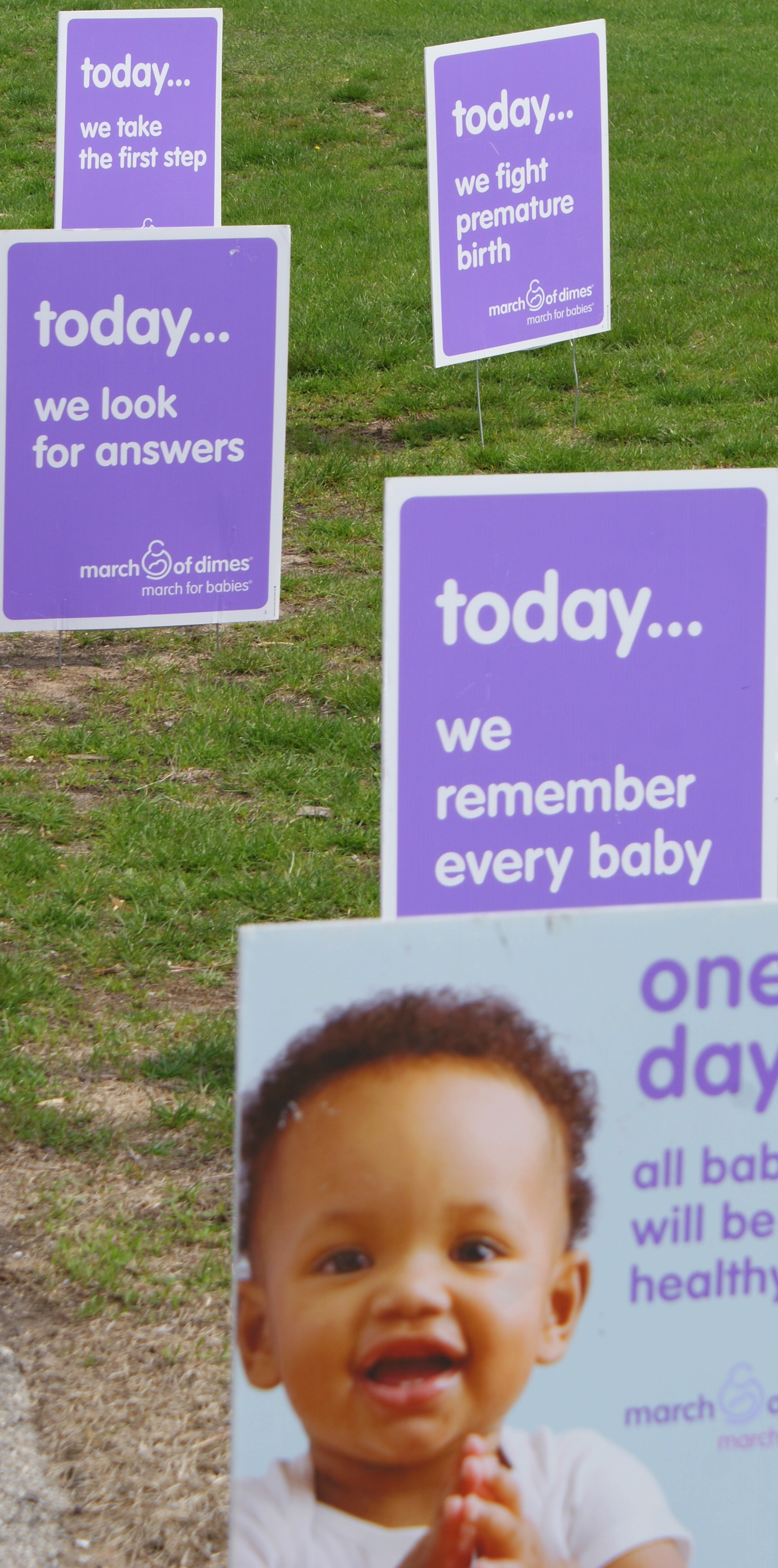This vertical photograph showcases a row of five yard signs arranged in a staggered formation, all aligned towards the camera. The signs are predominantly purple with white text, except for the closest one in the foreground. 

Starting from the background, the furthest sign reads, “Today we take the first step.” The second sign proclaims, “Today we fight premature birth.” The third sign states, “Today we look for answers.” The fourth sign declares, “Today we remember every baby.” 

The foreground features the closest yard sign, which prominently displays an image of a young Black baby or toddler. There is text in purple on the right side of this sign, but it is partially cropped off and not entirely legible.